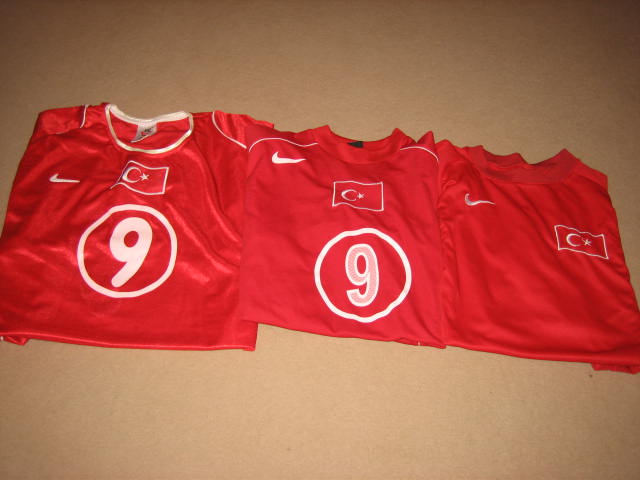The photograph captures three red sports jerseys, neatly folded and arranged horizontally against a beige backdrop. Each jersey, predominantly red with white accents, features the Nike swoosh logo on the top left. Central to the design is a white square with a crescent moon and star, reminiscent of the Turkish flag, though their placement varies across the jerseys. The two jerseys on the left prominently display a number nine within a white circle, with slight differences in font and transparency. The leftmost jersey also stands out with a white ring around the neck and shoulders, while the middle jersey has a thin white stripe along the shoulder lines. The rightmost jersey lacks the number nine but shares the same glossy, silky polyester material of the others. The jerseys partially overlap each other, enhancing the cohesive yet varied design elements, all beautifully illuminated with a gradient lighting effect on the backdrop.